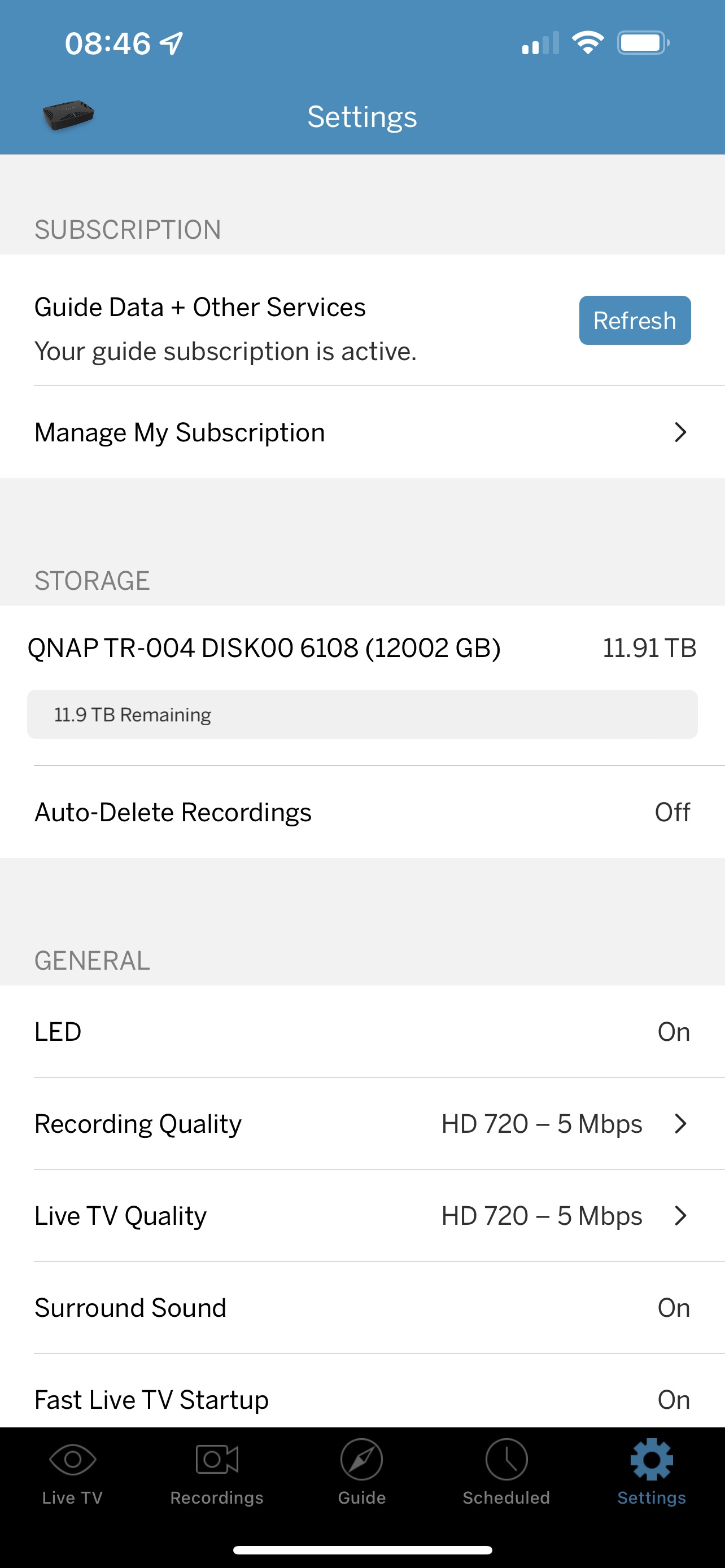The image displays a user interface centered around a subscription and storage management system. Starting from the top, there is a dark blue border showing the time as 8:46, two network bars, and an almost full battery icon. Directly beneath, the header reads "Settings" in white text.

Below the header, there is a gray section labeled "Subscription" followed by a white section detailing that the user's guide subscription is active, accompanied by a blue "Refresh" button and another option labeled "Manage My Subscription."

Further down, another gray box titled "Storage" is present. Within this section, white text displays details of a storage device: "QNAP TR-004 DISK-006108" with a total capacity listed as "12002 GB" and "11.9 TB." The remaining space is noted as "11.9 TB". 

Following this, there's an indication of "Auto Delete Recording: Off." Finally, another header labeled "General" below which the setting "LED: On" is displayed.